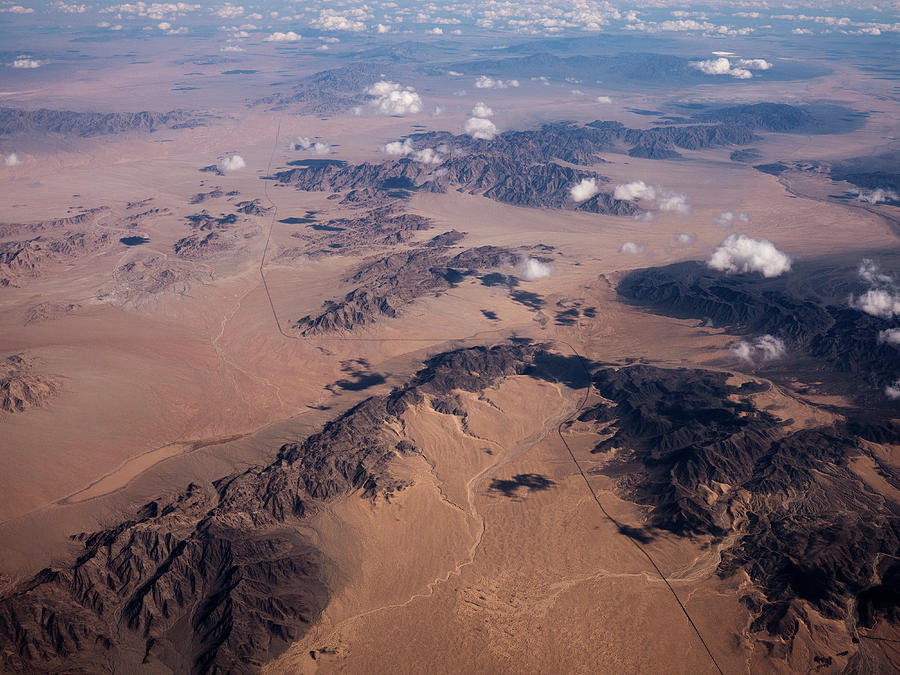This high-altitude aerial photo showcases a vast, extremely dry desert landscape interspersed with rugged hills and dark brown, almost blackish cliffs. The ground is arid and barren, devoid of any green vegetation, conveying the harshness of the terrain. Dried-up riverbeds snake through the land, suggesting where water may have once flowed, while a possible road or man-made structure cuts through the flatter areas, avoiding the more elevated sections. The entire landscape is speckled with light cloud cover, with the density of clouds increasing toward the top of the image, making the overall hue lighter in that section. The perspective from above the clouds provides a unique vantage point, emphasizing the desolate and expansive nature of the desert below.